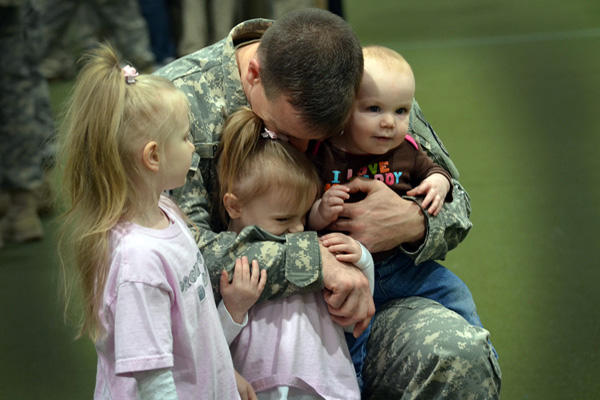In this poignant color photograph, a military father, dressed in standard Army fatigues, is kneeling on his right knee while tenderly embracing his three young children, all of whom have fair skin and long blonde hair in ponytails. The scene has a greenish hue due to the olive drab wall in the background, illuminated by a light that casts a gentle glow on the family. The youngest child, a boy of about one year old, is perched on his father's knee, wearing a brown "I Love Daddy" shirt and blue pants. The father holds him close with one arm, perhaps kissing the top of his head. The middle child, a girl likely around three or four years old, clings tightly to her dad’s other arm, wearing a pink t-shirt and looking comforted by his embrace. Standing slightly apart but watching lovingly is the eldest daughter, who appears to be about six or seven and is also wearing a matching pink shirt. In the background, the lower limbs and combat boots of other military personnel are visible, creating a stark contrast and adding depth to the emotional moment captured.